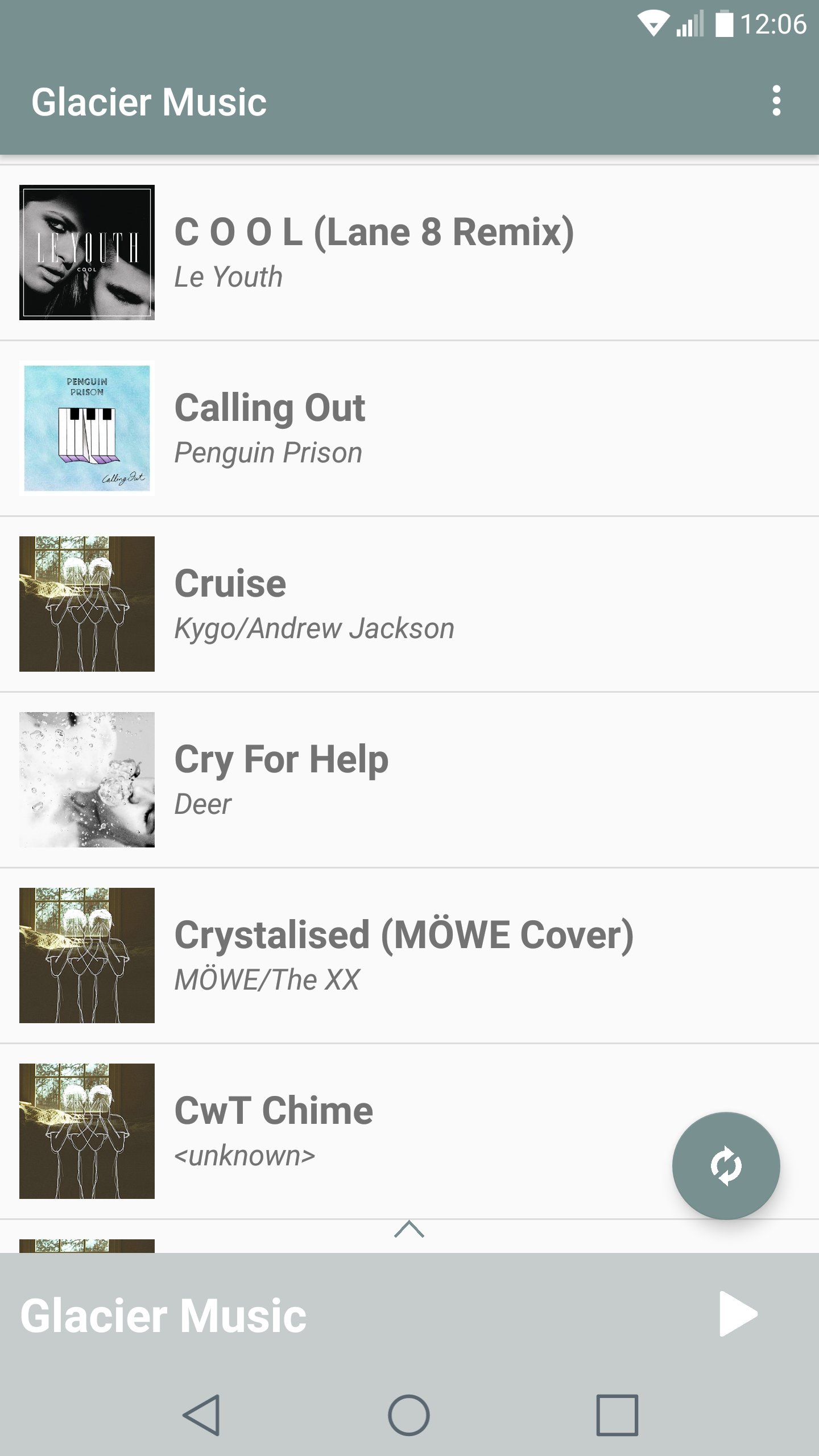This image shows a webpage displayed on a smartphone, provided by Glacier Music, as indicated by the white text in the top bluish rectangle of the screen. The time reads 12:06 in the top right-hand corner, with icons for battery power and signal strength next to it. On the left, there are three clickable dots that open a menu of options. 

Below this header, there's an image of a band called Kool, with the text "Lane 8 Remix La Youth." Following that, we see another band's album cover titled "Calling Out" by Penguin Prison. 

Next, there's an album cover labeled "Cruise," featuring the artists Kygo and Andrew Jackson. Below this, another album cover appears, titled "Cry For Help," with text that might refer to the song "Dear" or suggest that "Cry For Help" is the track and "Dear" is the band.

Further down, there is a song named "Crystallize" with a cover by Mo featuring The XX, accompanied by the text "CWT Chime" and a note indicating "Unknown" for the band name.

At the bottom of the webpage, the Glacier Music logo is displayed again, accompanied by three symbols: a triangle, a circle, and a square.